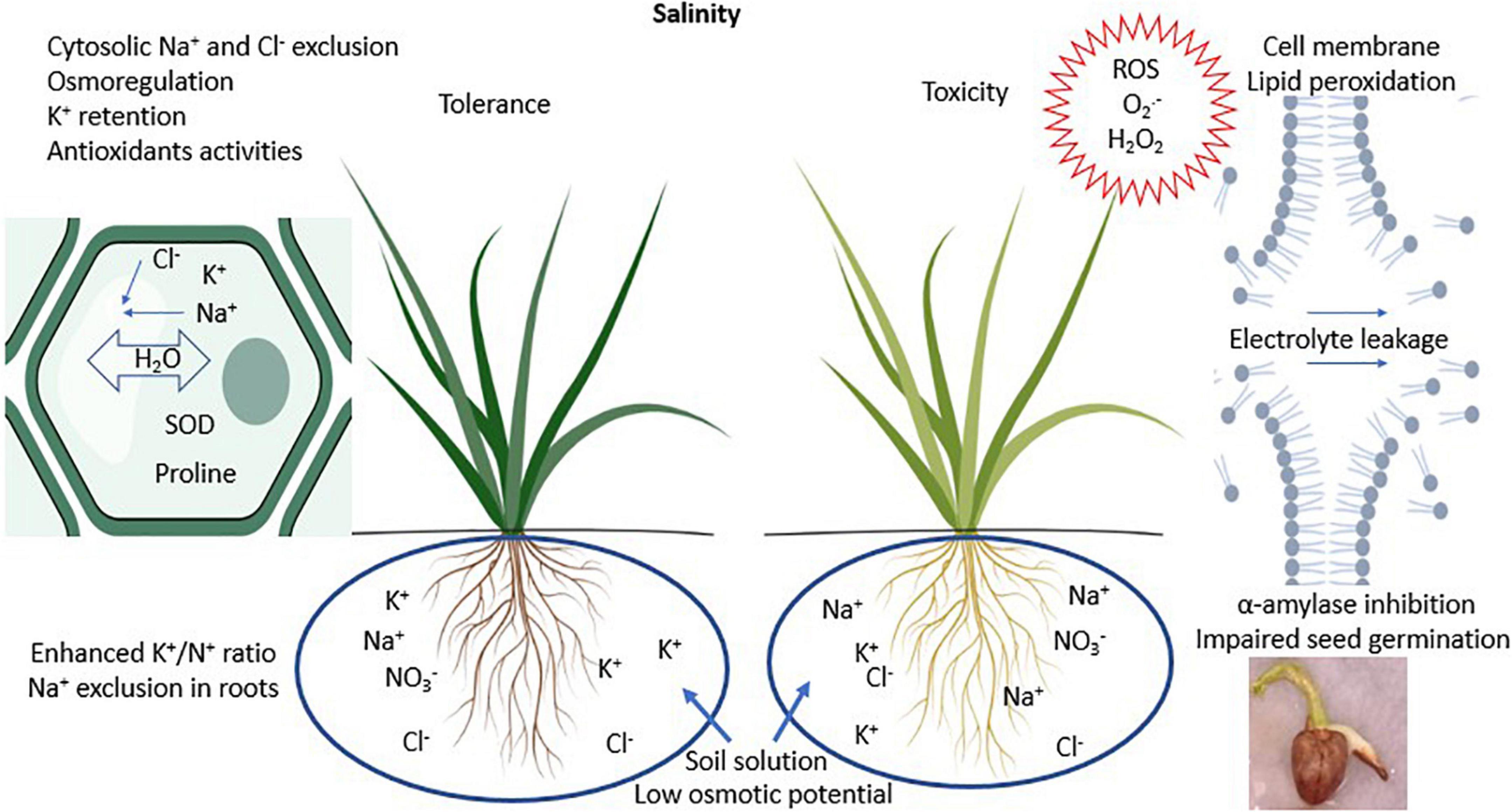The diagram, set against a white background, presents an in-depth explanation of the effects of salinity on plants, specifically focusing on tolerance and toxicity. At the top center, the word "Salinity" is prominently displayed. Directly beneath, two centered headings labeled "Tolerance" and "Toxicity" each display an illustration of a plant with green leaves sprouting from blue circles representing the roots. The "Tolerance" side features dark green leaves and a detailed depiction of the roots containing potassium ions, sodium ions, nitrate ions, and chloride ions. In contrast, the "Toxicity" side shows lighter green leaves with roots containing sodium, potassium, and chloride ions, and a similar presence of nitrate ions. 

Between these two root illustrations, the phrase "Soil solution, low osmotic potential" appears, with two blue arrows pointing towards the respective blue circles. The left side of the diagram highlights "Cytosolic sodium and chloride exclusion, osmoregulation, potassium retention, antioxidant activities" alongside a smaller diagram. Further down on this side, text indicates "Enhanced potassium/nitrogen ratio, sodium exclusion in roots."

On the upper right side, the title "Cell membrane lipid peroxidation" is accompanied by a diagram illustrating "Electrolyte leakage" with arrows and “Alpha amylase inhibition, impaired seed germination” in the lower right corner. This section vividly illustrates the detrimental effects on plant cells, completing the diagram's detailed portrayal of how soil salinity affects plant growth and physiology.